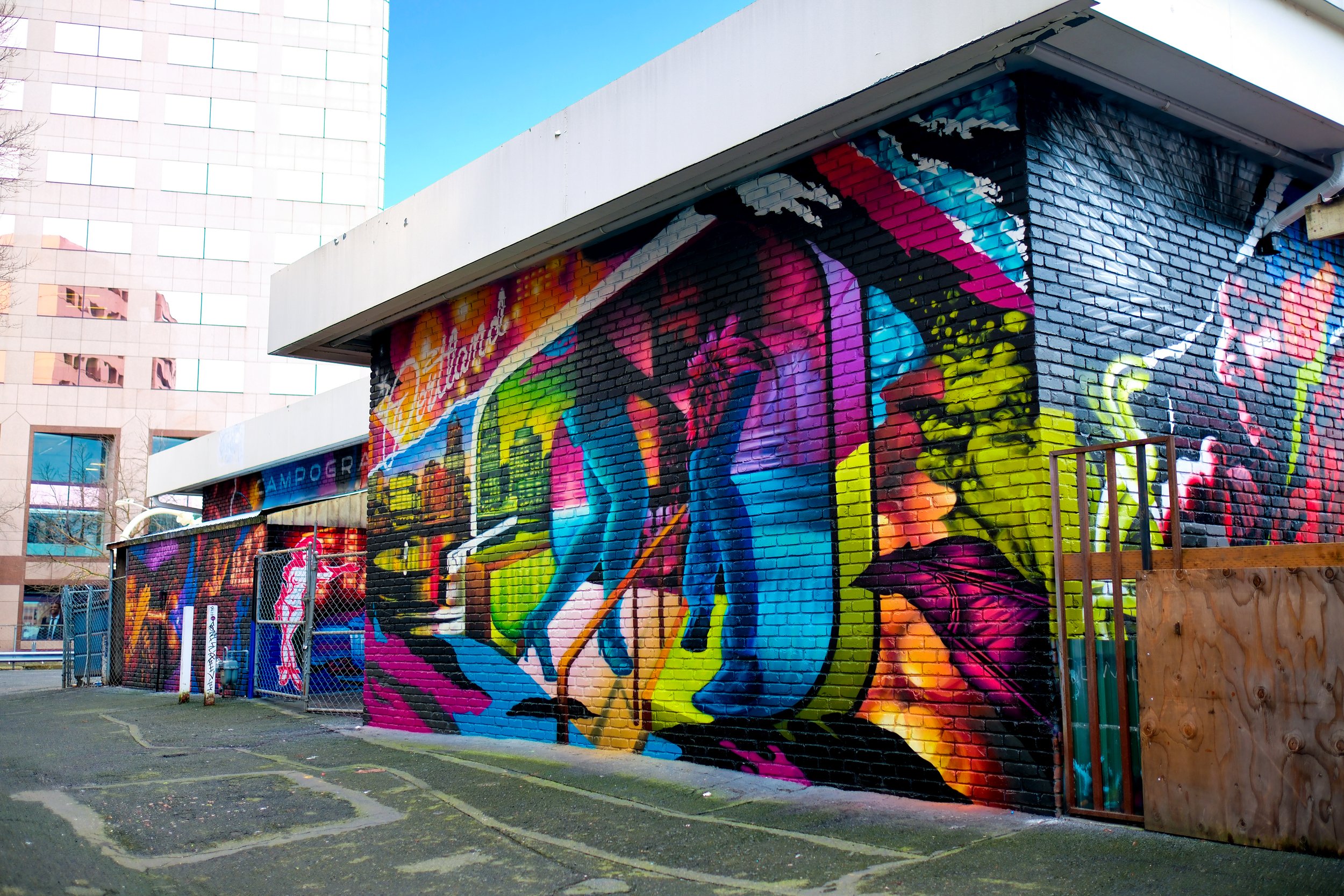This daytime photograph, rectangular in shape (6 inches wide by 3 inches high), captures an urban scene accentuated by vibrant street art. In the lower left corner, a paved walkway, noticeably patched with light and dark gray concrete, leads diagonally to the right. Dominating the middle of the image, side-by-side square brick buildings emerge with their bricks painted in vivid hues. On the building to the left, whimsical paintings of dancing figures in bright purple, blue, green, and orange hues adorn the brick facade. The artwork prominently features the legs of a man and woman in blue jeans, appearing to dance amidst a colorful cityscape in the background, which includes yellow buildings.

In the upper left corner, the building displays "Portland" written in white cursive. Adjacent to this building, another structure features a painted image of a mostly nude woman with red hair and a red bikini. Separating the two buildings is a metal gate. Both building roofs are flat and gray.

On the right side of the image, a plywood wall, possibly serving as a makeshift barrier, stands out. To the left side, a tall stone skyscraper reaches up, touching a patch of blue sky peeking through the urban landscape, juxtaposing the smaller, colorful buildings in the foreground. The artistic facade sits across from this towering office building, hinting at a parking lot or asphalt area around it.